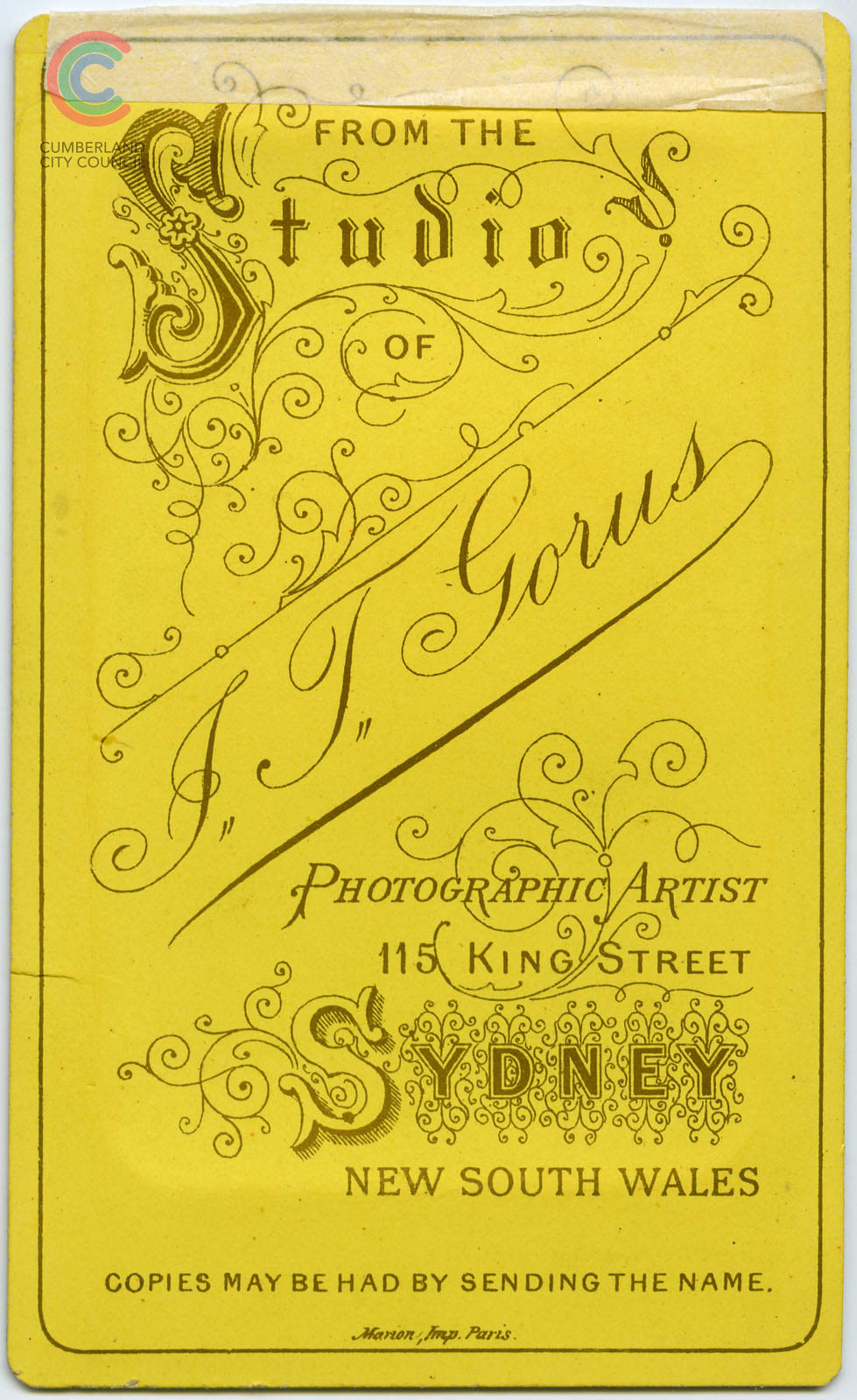This image is a vertically-hung rectangular poster with a bright yellow background and black typeface. In the top left corner, there's a conspicuous multicolored triple-C design: the outer C is red, followed by green, and finally blue. Just below this is the text "Cumberland City Council." The central portion of the poster features ornate, scroll-like calligraphy. It reads, "From the studio of A.J. Gorus," diagonally from the bottom left to the top right, with "studio" adorned with intricate flourishes. Underneath, it's labeled "Photographic Artist, 115 King Street, Sydney, New South Wales." The bottom part of the poster states, "Copies may be had by sending the name Marion Impression Paris," with more decorative scrollwork interspersed throughout the design, giving it an old-fashioned, vintage appearance.